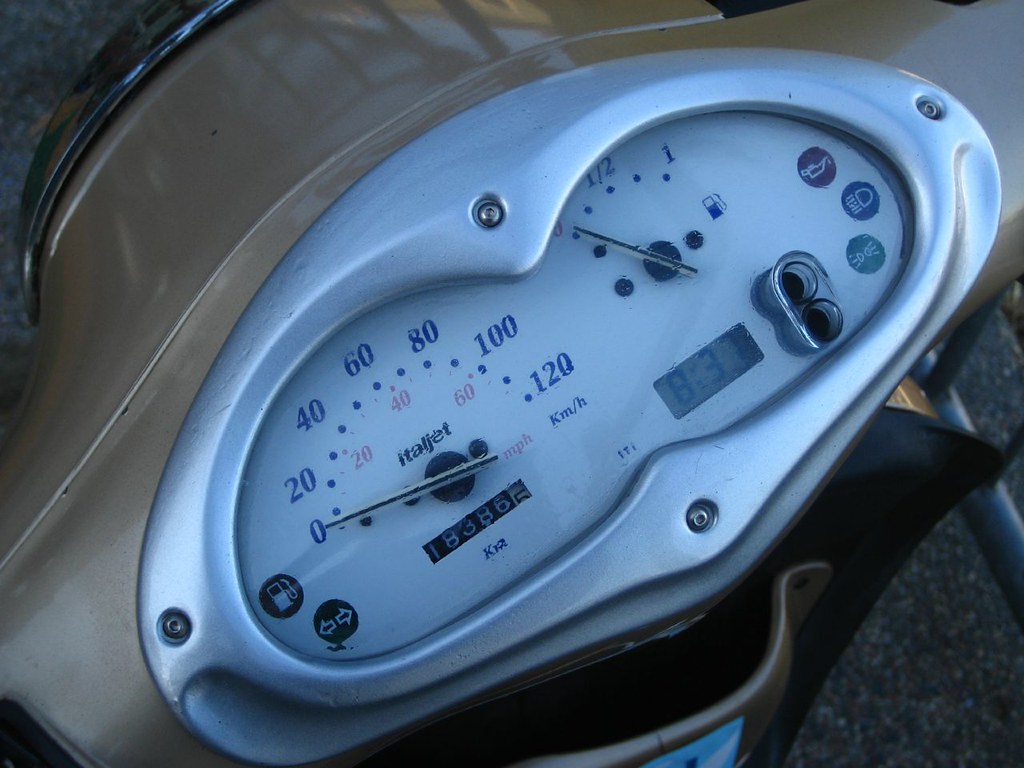This is a vibrant color photograph capturing a close-up view of a scooter's control panel. Encased in a sleek, silver, and shiny casing, the panel prominently displays various gauges and indicators. The scooter behind the panel appears to be painted in a rich brown color. On the left side of the control panel is the speedometer, with its needle resting at zero and speed increments marked up to 120 km/h. The brand name "ITALJET" is clearly inscribed in the center of the panel. Below the brand name, the odometer reads 18386, on the verge of ticking over to 18387. To the far left is a versatile gauge that includes both a gas level indicator—marked from zero, through half, to full—and a left-right turn signal indicator.

On the opposite side of the panel, additional indicators can be found. The gas gauge is set at zero, next to a small icon of a gas pump. There's also an LCD screen displaying the number 837. The control panel’s casing has some visible wet spots, indicating either recent use or weather conditions. To the right, icons for oil levels, headlights, and high beams are clearly visible, offering vital information to the rider. This detailed image showcases the scooter’s well-maintained and intricate control features, reflecting both functionality and design.